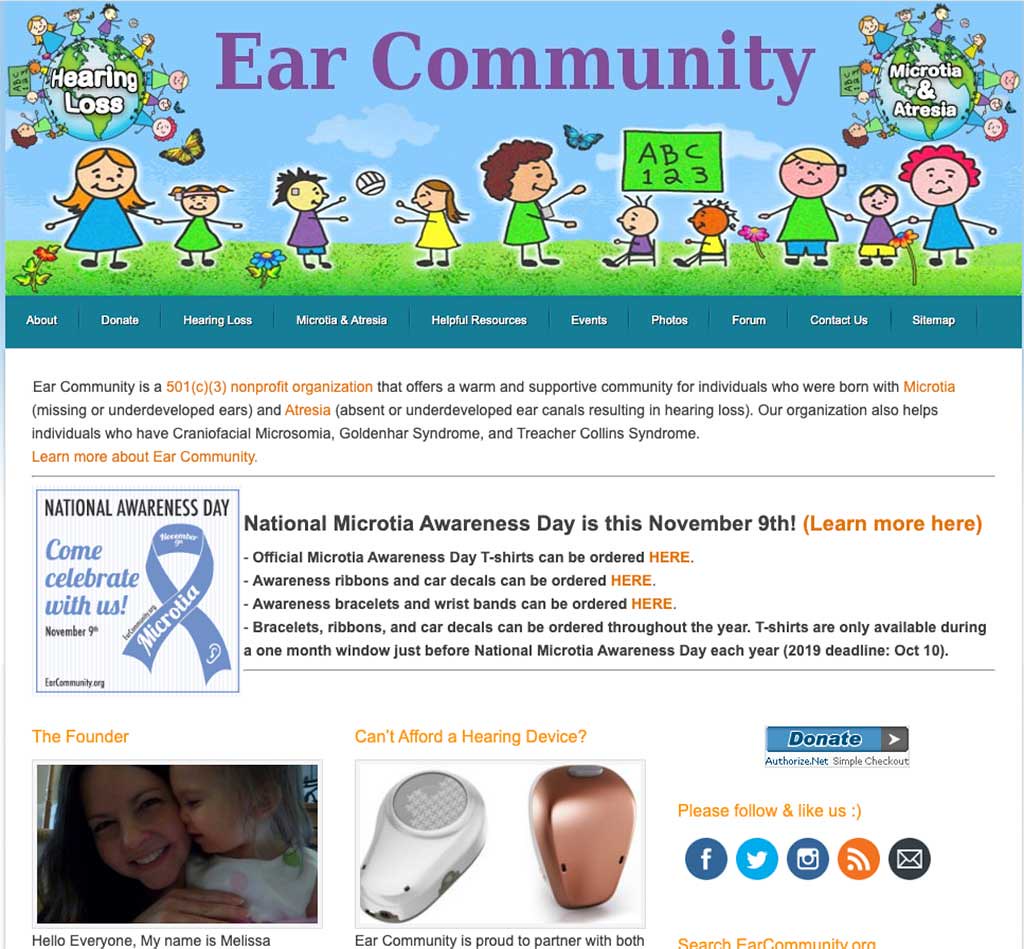The image depicts a vibrant webpage for the "Ear Community" organization, which is distinctly designed with a blue background and purple text at the top. The header reads "Ear Community" and is accompanied by cheerful cartoon drawings of children and adults playing on green grass, surrounded by butterflies and flowers, creating a warm and inviting atmosphere. On the top left and right corners, there are globes with children holding hands around them. The left globe reads "Hearing Loss," while the right one reads "Microtia and Atresia."

Below the header, there are several navigation tabs including "About," "Donate," "Hearing Loss," "Microtia and Atresia," "Helpful Resources," "Events," "Photos," "Forum," "Contact Us," and "Sitemap." Prominently featured below these tabs is a text block describing Ear Community as a 501(c)(3) non-profit organization dedicated to supporting individuals born with microtia (missing or underdeveloped ears) and atresia (absent or undeveloped ear canals), both resulting in hearing loss. The organization also extends its support to individuals with craniofacial microsomia, Goldenhar syndrome, and Treacher Collins syndrome.

Further down, there's a banner highlighting awareness days, with additional details about National Microtia Awareness Day in November. The bottom left of the page showcases a photo of the founder alongside her child, emphasizing the personal and compassionate nature of the community. At the bottom center, images of hearing aid devices are displayed with a call-to-action in yellow text that reads, "Can't afford a hearing device?" The bottom right corner is filled with various social media posts, rounding out a comprehensive and interactive website devoted to ear-related conditions and support.